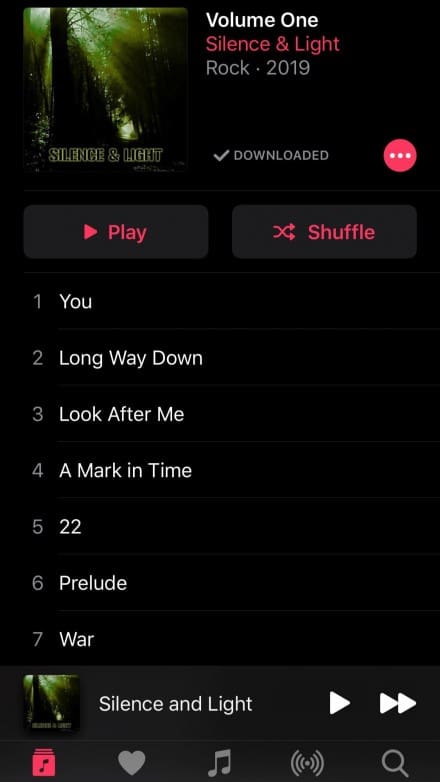On a black background, the screen resembles that of a mobile music player. At the top is an album cover image displaying the text "Silent and Night," underneath which it reads "Volume One: Silence and Light - Rock 2019." The album has been marked as downloaded and checked. To the right of the album cover is a round red button with three vertical dots, indicating additional options.

Below this section are the playback buttons: a play button and a shuffle button, both with red font on dark gray buttons. A tracklist follows, listing the songs included in this album:

1. Silent
2. Long Way Down
3. Look After Me 
4. A Mark in Time
5. 22
6. Prelude
7. War

At the bottom, another banner features the same album cover image on the left, with the text "Silence and Light" in white next to it. This section includes a white play button and a white fast-forward button. Adjacent to this is a square icon featuring a black music symbol.

The bottom menu bar is gray and contains several icons in gray: a heart, a music note, a Wi-Fi or broadcast symbol, and a magnifying glass for search. The album cover also incorporates some green elements, standing out against the predominantly dark theme.